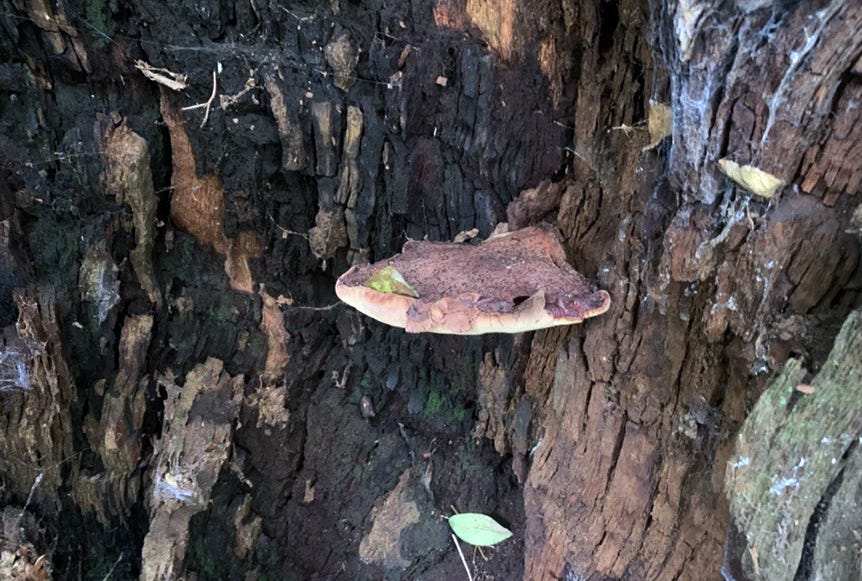The image depicts a close-up view of an aged and weathered tree bark, which exhibits a range of colors including traditional brown, dark black, and portions that appear white, possibly due to spiderwebs or sticky white sap. The bark has an old, possibly burnt appearance, hinting at past damage, perhaps from a forest fire. On the right-hand side, delicate spiderwebs are visible, suggesting the presence of spiders living underneath the bark. Centrally featured is a prominent brownish, rounded object that resembles a mushroom or fungus. Its structure is flat and triangular, with light beige coloration on the underside and a darker brown on top. This mushroom fungus, seemingly non-edible and likely poisonous, protrudes from the tree, adding an intriguing element to the naturally intricate landscape of the tree's bark. Additionally, a solitary green leaf rests on the fungous growth, further highlighting the scene's detailed and textured complexity.